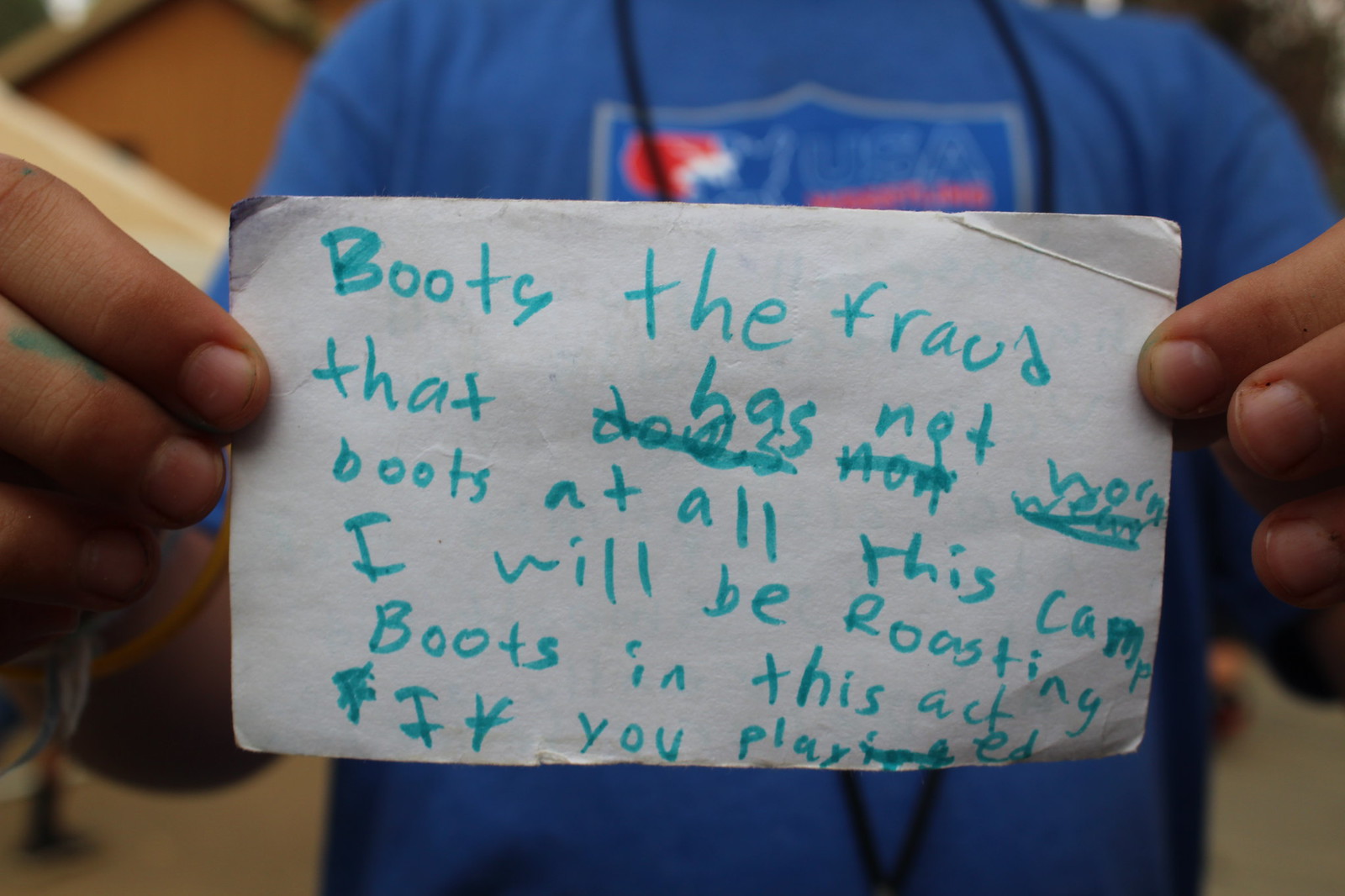This horizontally aligned rectangular image features a middle-school-aged child, dressed in a blue T-shirt, holding a small, worn index card. The child, whose face is not visible in the image, has short nails and slightly ink-stained fingers from a blue marker. The background is blurry, revealing only the upper body of the child against a white backdrop. The handwritten note on the card, penned in blue marker, has words and phrases that are somewhat difficult to decipher due to crossed-out sections, childlike handwriting, and possibly being written in a hurry. The note reads, "Boots, the fraud that has not worn boots at all this camp. I will be roasting Boots in this act if you played." This peculiar message appears to reference an inside joke or a playful event at camp revolving around someone named Boots who notably hasn't worn boots, suggesting a light-hearted competition or performance.